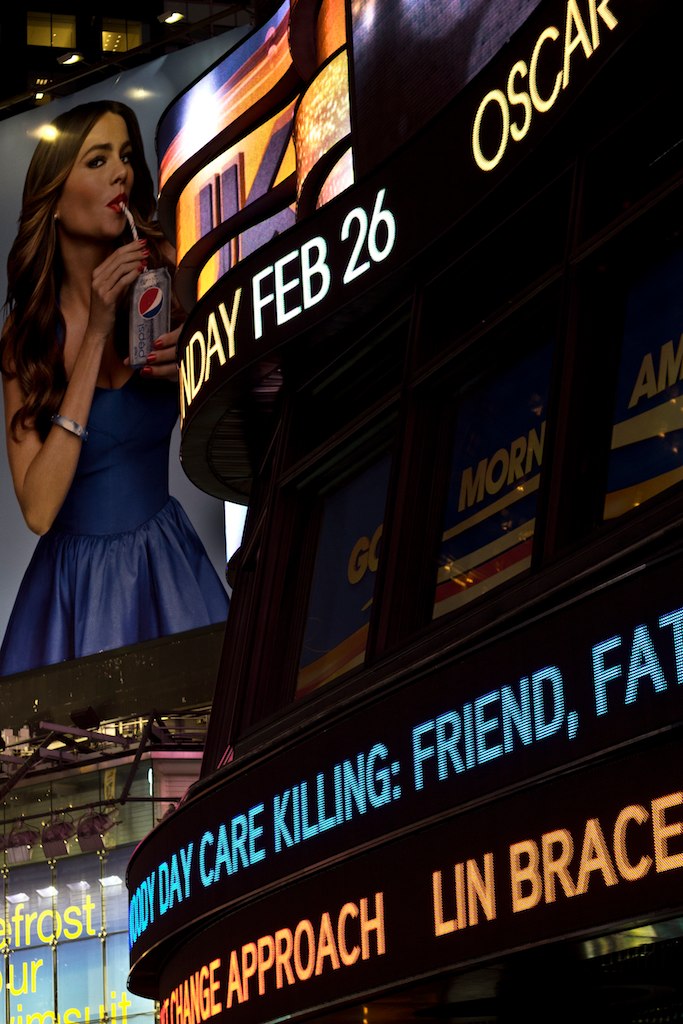This detailed outdoor color photograph captures the facade of a building from street level, prominently featuring a large digital marquee and vibrant billboard elements. In the lower right, two digital marquee bands in orange lettering partially display the words "approach" and "L-I-N-B-R-A-C-E." Above this, another marquee cryptically reads "daycare killing; friend, F-A-T." Dominating the upper right corner is a large display poster of actress Sofia Vergara. She is wearing a sleeveless blue dress, sipping from a silver Diet Pepsi can with a straw, her face in a three-quarter view. Her long brunette hair cascades down as she raises her right forearm to hold the straw. Adjacent to this display, a digital marquee in white letters shows the date "FEB 26," and extending out of the frame is part of the word "OSCAR." The upper right portion of the photograph also hints at another sign or lighting from an adjacent storefront, suggesting this scene is set in a bustling urban area, possibly an entertainment complex.